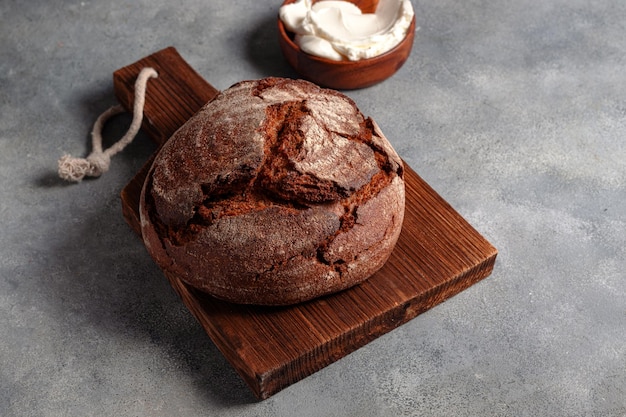The image showcases a meticulously baked, artisanal loaf of bread resting on a dark brown wooden pizza paddle. The loaf is a deep, dark brown color, reminiscent of pumpernickel or rye bread, with rustic imperfections and splits from the baking process. A light dusting of white flour sprinkles the top of the round loaf, adding to its handcrafted appearance. The pizza paddle, elegantly dark wood, features a beige rope threaded through a hole at the top, enhancing its rustic charm. In the background, the photograph is set against a gray, two-toned marble-like surface. A small, round wooden bowl sits nearby, containing a pat of creamy white butter, adding a touch of indulgence to the scene. The artisanal sensibility is further emphasized by a piece of white fabric or towel tucked into the bowl, hinting at the homely, crafted nature of the bread's presentation.